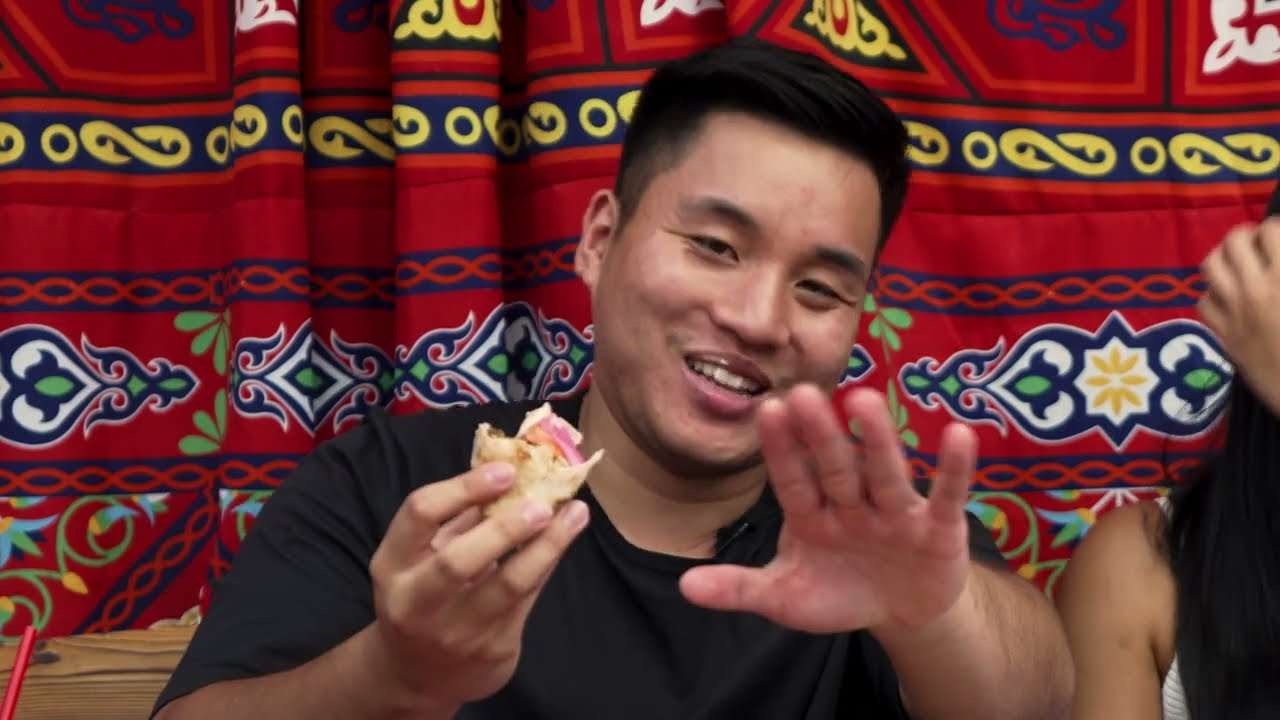This image captures a candid moment featuring a smiling man of apparent Asian descent, wearing a black t-shirt, and holding a piece of food, possibly a sandwich or pastry, in his right hand. Some of the food is visible on his upper lip. His left hand is raised with the palm facing the camera, as if playfully resisting the photograph. The man has dark hair and short haircut. Seated next to him on his left side is a woman, partially visible in the frame, wearing a white tank top and possessing dark, possibly brown or black hair. Behind them hangs an eye-catching red curtain adorned with a variety of tribal-inspired patterns: blue stripes with yellow infinity symbols, and intricate floral designs in bright colors like yellow, blue, white, green, and turquoise. A brown table also appears in the lower background with a straw visible in the lower left corner.